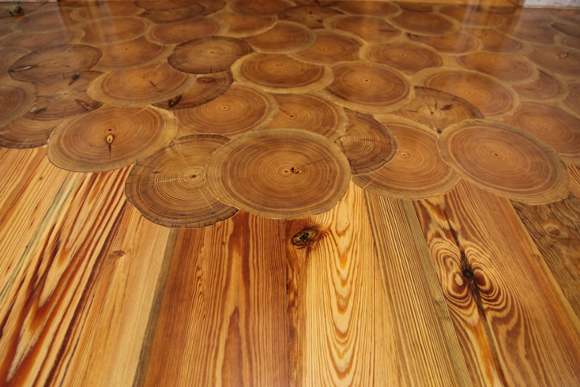This color photograph showcases a highly polished wooden surface, possibly a floor or countertop, viewed at a slight angle. The lower part of the image features long, straight, and heavily grained wooden boards in a light pine tan color with various knots, suggesting a simple and clean aesthetic. As the eye moves upward, the surface transitions to an intricate pattern of overlapping wooden discs, resembling thinly sliced log rounds or frisbees of wood. These discs, made from yellowish umber-toned timber, are laid out in a layered, intermingled fashion, creating a textured and visually engaging layout. The entire surface has been meticulously smoothed and sealed, likely with multiple coats of polyurethane, giving it a glassy finish that reflects the camera's flash. The photograph gives a sense of a well-crafted, beautiful piece, evoking both rustic charm and refined craftsmanship.